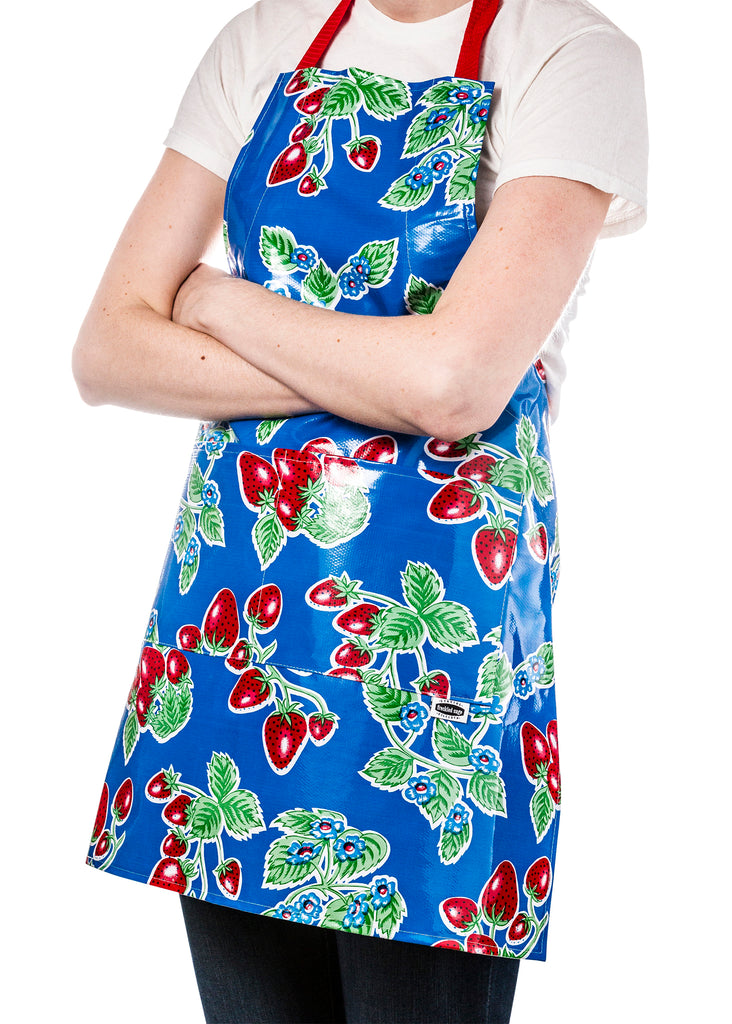The image depicts a Caucasian woman standing in a portrait orientation, with her head and legs out of frame, showing only from her shoulders to just above her knees. She is wearing a light cream-colored short-sleeved T-shirt and dark-colored jeans. Draped over her attire is a vibrant royal blue apron adorned with clip art-style strawberries, complete with green leaves and small blue flowers scattered throughout. The apron features a red neck strap and has a shiny, waterproof appearance, likely made of nylon or a similar material. The woman stands with her arms crossed in front of her, and the bright white background accentuates the vivid colors of her outfit, giving the scene a summery vibe.